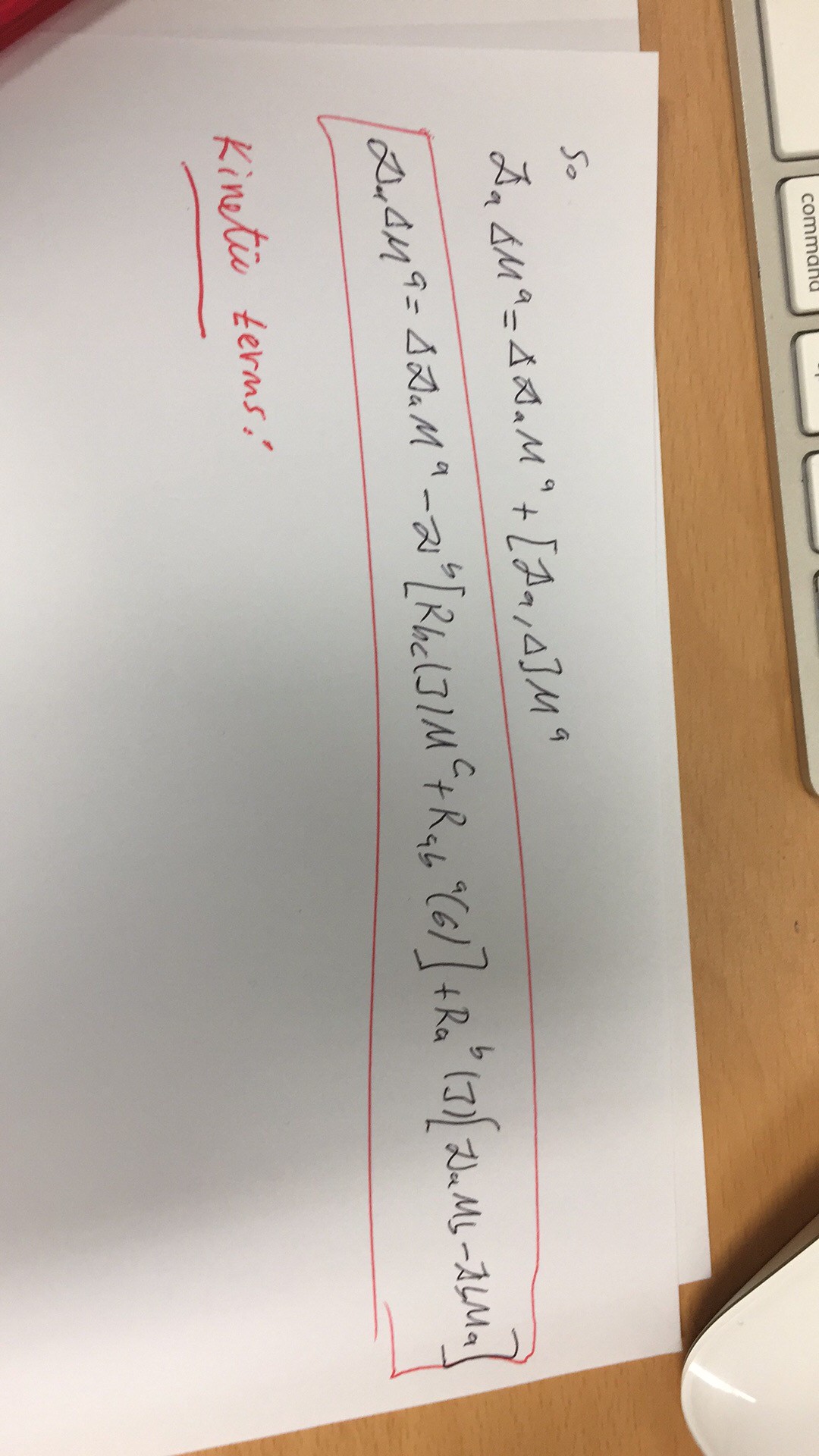The image captures a close-up view of a white sheet of paper placed diagonally on a wooden desk. Partially visible in the frame are the white and gray keys of a keyboard and the edge of a white computer mouse, emphasizing a workspace setting. The focal point of the photograph is the chemical reaction formula, meticulously inscribed in black ink on the paper. There are two distinct lines of chemical formulas, with the second line being notably longer than the first. This second line of the formula is distinctly highlighted with a red rectangle, drawing attention to its importance. Further emphasis is added by the handwritten annotation "kinetic terms" in red ink situated directly below the second formula line. The image, oriented sideways, provides a detailed glimpse into a moment of scientific notation and study.